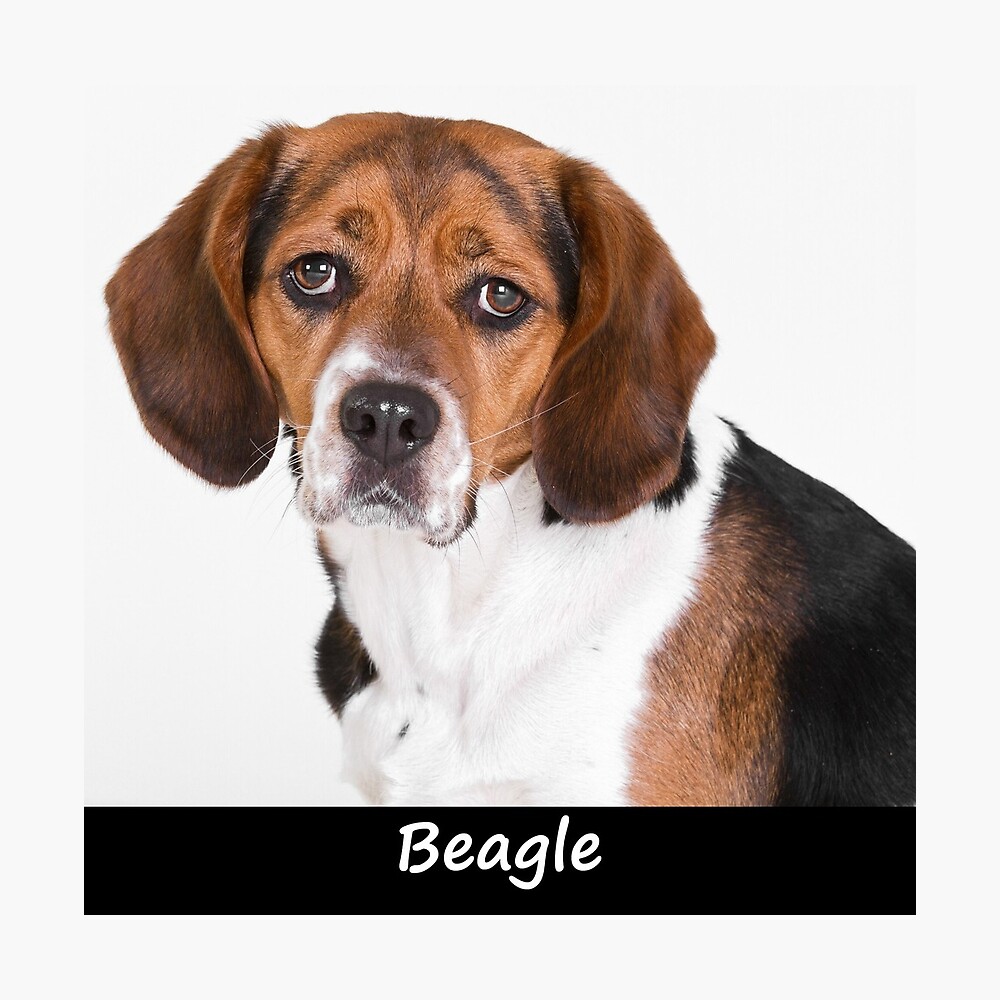This image features an adorable yet somewhat unhappy-looking young beagle, prominently centered against a light gray solid background. The dog's expressive dark brown eyes and black nose are framed by its brown and white snout, from which distinctive white whiskers protrude. The beagle's floppy ears add to its endearing appearance. Its fur is short and silky, with a captivating tri-color pattern: a primarily white neck and chest that transitions into a brown midsection and almost black back. Above the beagle's eyes, two distinct markings add character to its face. At the bottom center of the image, the word "Beagle" is displayed in white letters with a capital 'B,' ensuring the breed's identification. Despite its cute features, the dog appears almost to be frowning, adding a touch of melancholy to its expression.